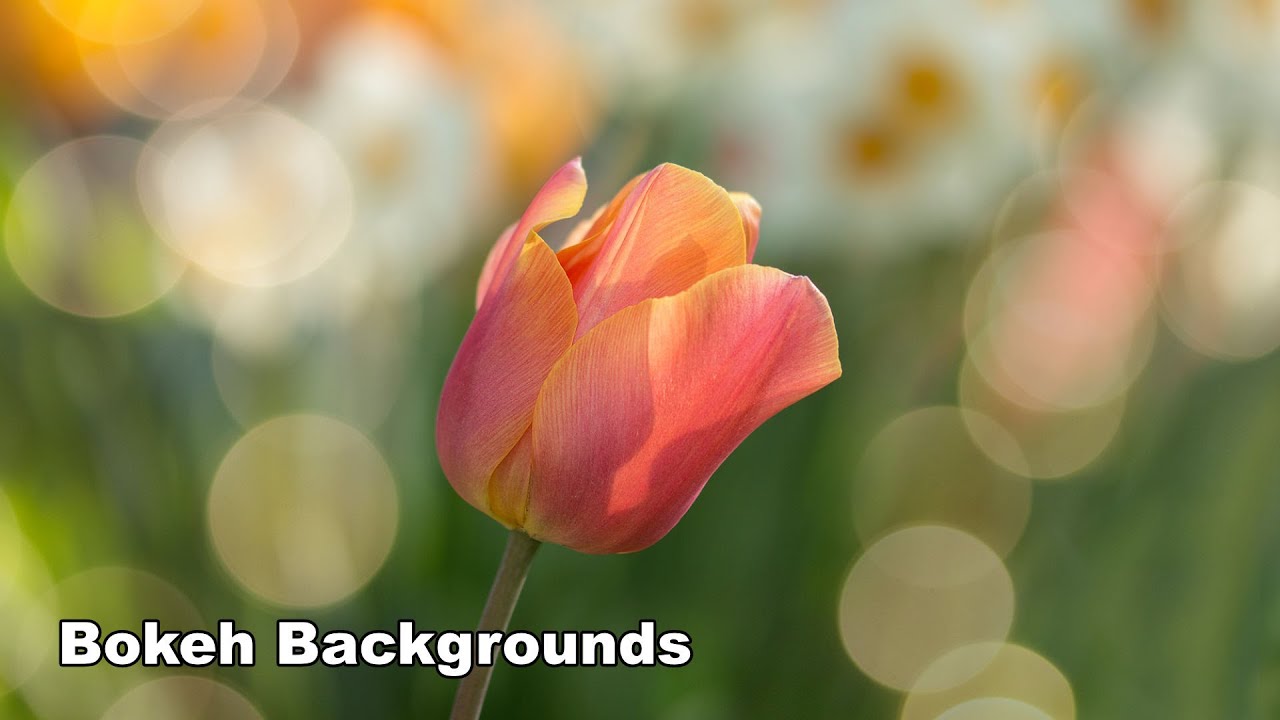This striking photograph captures a vibrant flower from a side perspective, showcasing its stunning details with a shallow depth of field. The flower, which closely resembles a tulip, boasts reddish petals with a hint of orange and yellow hues, tightly clustered together in layers rather than fanning out. The background is out of focus, resulting in a dreamy bokeh effect characterized by diffused green tones and light circles, which contrasts beautifully with the flower's vivid colors. Notably, the stem of the flower appears grey. The lower left corner of the image features white text with a dark border, displaying the words "bokeh backgrounds."